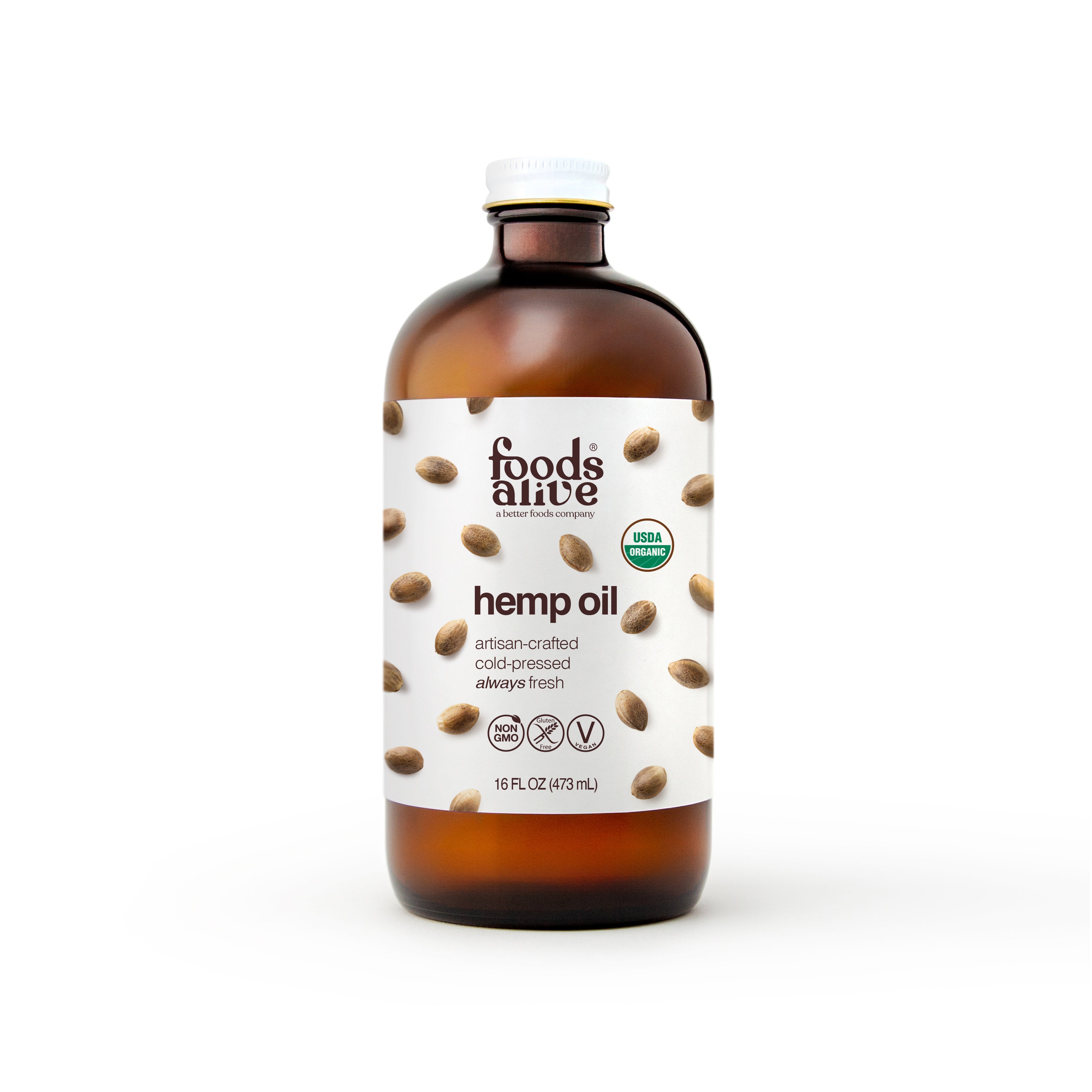This image depicts a 16-fluid ounce (473 milliliters) amber glass bottle of hemp oil from the brand Foods Alive. The bottle features a white metal screw-on cap and a white label adorned with brown hemp seeds. Prominently displayed at the top of the label, "Foods Alive" is printed in brown, and to the left, there is a green and white USDA Organic logo. Below the "Hemp Oil" title, the label reads "Artisan Crafted, Cold Pressed, Always Fresh." Additionally, towards the bottom, there are three distinct logos: one for Non-GMO, and others indicating gluten-free and vegan. The overall presentation is set against a clean, white background.